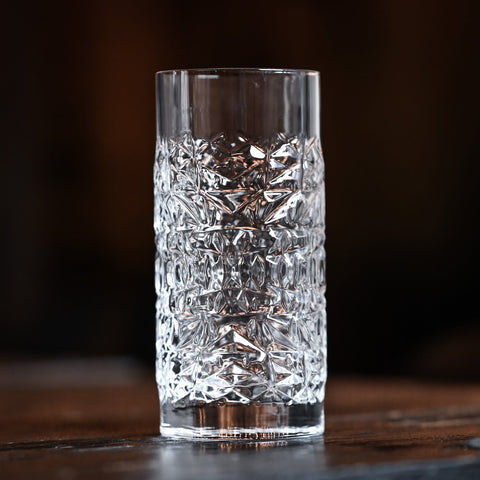The photograph features an empty drinking glass prominently positioned in the center of the frame, resting on a dark, slightly out-of-focus wooden table. The glass, pure and crystal clear, holds about 8 ounces and showcases an intricate decorative pattern resembling ice crystals. This frosted pattern begins approximately half an inch from the bottom and extends up to an inch below the rim, making it less transparent in that section. The background is a deep black, further drawing attention to the glass and its unique design. Potentially captured in a bar setting, a kitchen, or as a stock image for a store, the overall composition emphasizes the elegant yet functional artistry of the water glass amidst the contrasting textures and colors of its surroundings.